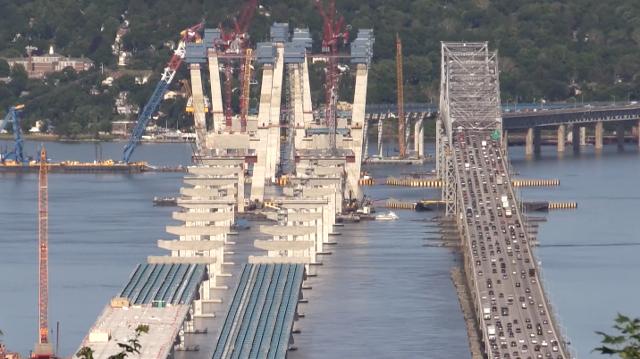In this detailed aerial photograph of a bustling city area, three distinct bridges span a large river. On the right side of the image, a finished bridge with at least six lanes accommodates heavy traffic, evidenced by the numerous cars densely packed across its span. This bridge slopes upward, seamlessly integrating into an extensive highway network. On the left, two separate yet closely positioned bridges are either under construction or demolition. The bridge frameworks, constructed from white concrete, indicate extensive ongoing work facilitated by a crane, with steel pieces visible in the water, likely waiting to be lifted into place. Beyond the river, a lush green mountain occupies the upper third of the photo, topped with numerous houses. The entire scene is captured from an elevated viewpoint, offering a comprehensive view of the bridges, the vast river, and the verdant hillside, perfectly illustrating the intersection of urban development and natural beauty.